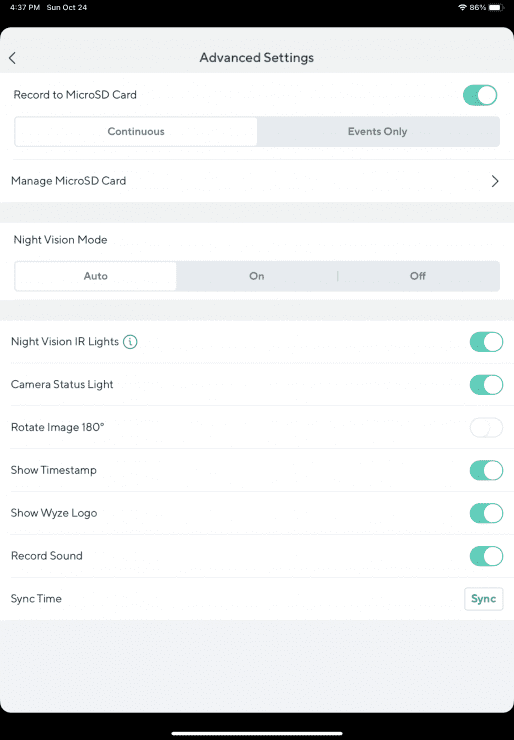Screenshot dated Sunday, October 24th at 4:37 PM, displaying a mobile device interface with a white background and an 86% battery level. The interface includes various settings within a gray rectangle:

- **Navigation Arrow**: Positioned on the left side.
- **Advanced Settings Header**: Clearly marked on the screen.
  
### Camera Recording Settings:
- **Record to micro SD Card**: Toggled ON.
- **Recording Mode**:
  - "Continuous" option highlighted in a white rectangle.
  - "Events Only" option in a gray rectangle.
  
### micro SD Card Management:
- **Manage micro SD Card**: Indicated with a right-hand arrow.

### Night Vision Mode Settings:
- **Night Vision Mode**: Situated in a blue rectangle.
- **Options**:
  - "Auto" in a white rectangle.
  - "On" and "Off" options in separate gray rectangles.
  
### Additional Settings and Toggles:
- **Night Vision IR Lights**: Displayed with a blue circle featuring a blue eye, toggled ON.
- **Camera Status Light**: Toggle bar ON.
- **Rotate Image 180 Degrees**: Toggle bar OFF.
- **Other Active Toggles**:
  - **Show Timestamp**
  - **Show WYZE Logo (W-Y-Z-E)**
  - **Record Sound**
  
### Synchronization:
- **Sync Time**: Accompanied by a gray rectangle with "Sync" in blue text.

### Bottom Interface Element:
- **White Bar** centrally located at the screen's bottom.